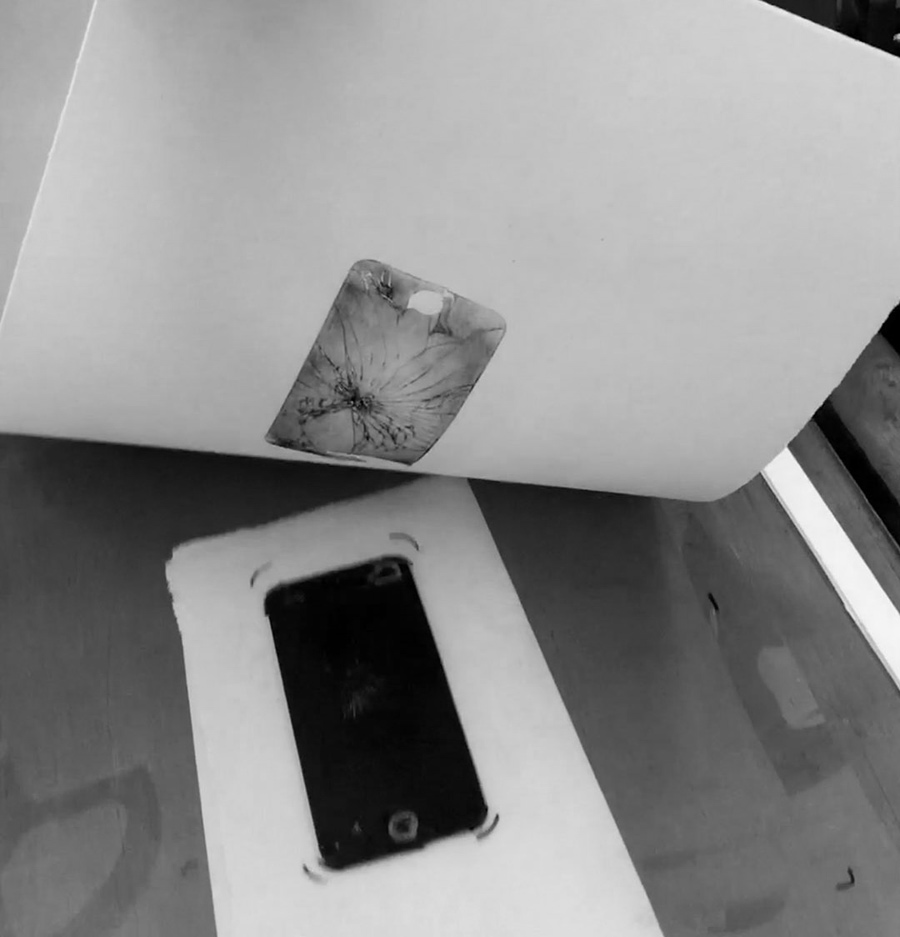This black and white photograph captures the top view of a copy machine-like surface with a metallic sheen. Centered at the bottom of the image is a rectangular white pad, upon which lies a smartphone's back. The smartphone features a prominent camera lens circle. Above the phone, a white sheet curves upward, suggesting motion, possibly implying the process of peeling or detaching. The surface layout hints at an additional feature: a sunburst-like etching that corresponds to the smartphone's dimensions. This might indicate that the phone and its cover were previously pressed together. The scene provokes curiosity about the events leading up to this precise arrangement, making the viewer question the exact circumstances captured here.